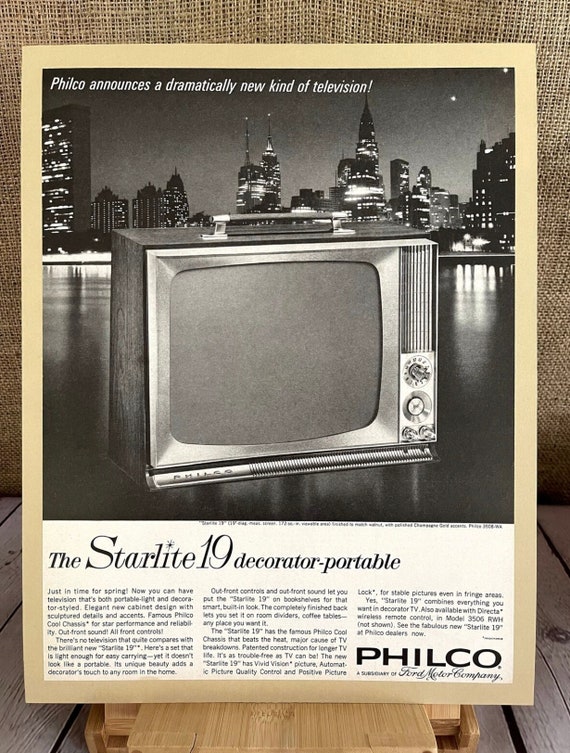In this image, a vintage black-and-white advertisement for a Philco television is displayed. The advertisement is mounted with a tan matting around the borders and situated on a wooden surface with a brown canvas background. The advertisement itself is divided into two sections. The upper section features an old television screen with a handle at the top, positioned over a river with a city skyline in the background. The skyscrapers are lit, suggesting it is nighttime. Above this image, the text reads, "Philco announces a dramatically new kind of television." The bottom section contains a detailed description of the television model, the Starlight 19 Decorator Portable. It highlights the TV's elegant new cabinet design with sculpted details and accents, and emphasizes its portability and decorative appeal. The text also notes the "Famous Philco cool chassis for star performance and reliability," and mentions features like out front sound and out front controls, which allow for versatile placement on bookshelves, room dividers, and coffee tables. The advertisement boasts the TV's vivid vision picture, automatic picture quality control, and positive picture lock. Additional features include direct wireless remote control available on model 3506 RWH. The Philco logo is prominently placed at the bottom right along with the note, “Philco, a division of Ford Motor Company.”